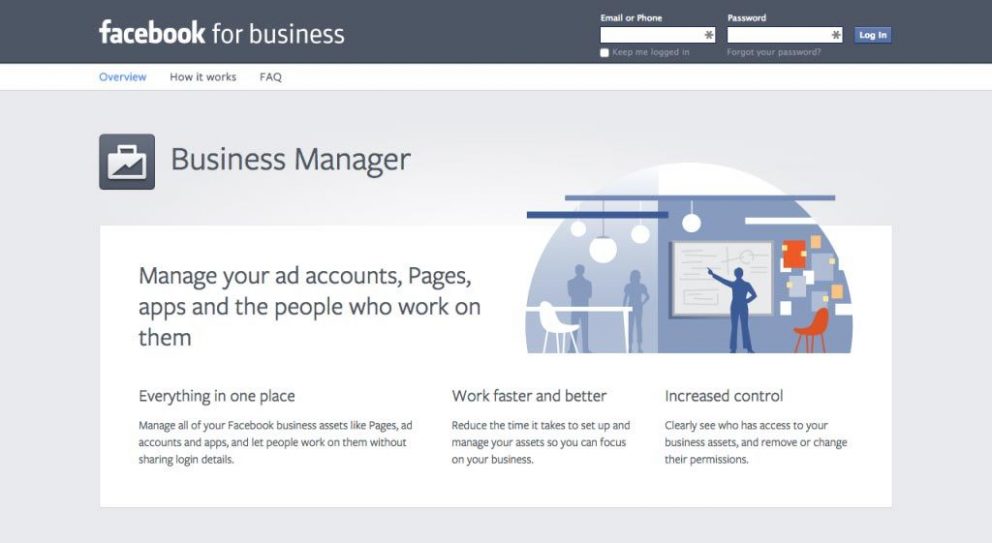A screengrab of Facebook Business Manager's login page is displayed prominently in the image. At the top of the page, we see the familiar "Facebook for Business" header, followed by fields where users can enter their email or phone number in a white rectangle. Below this, there is a password field. These sections are accompanied by essential buttons and options such as "Login," utilizing a star-shaped icon for emphasis, a checkmark box labeled "Keep me logged in," and a link offering to help those who "Forgot your password."

Directly below, the page provides navigational breadcrumbs including options like "Overview" and "How it Works." On one edge, a square icon introduces users to additional features, marking the start of an informative section. Here, we observe a briefcase icon followed by the heading "Business Manager."

In the center of this section, bold text highlights the primary functionalities: managing "Ad Accounts," "Pages," "Apps," and tracking "How many people work on them." A detailed subtitle further clarifies that everything is managed "In One Place," stating, "Manage all of your Facebook business assets such as Pages, Ad accounts, and Apps without sharing login details."

The description continues to emphasize efficiency, noting how users can "Work faster and better," and "Reduce the time it takes to set up resources so you can focus on your business." A tooltip-like detail points out how "Increase control" allows users to clearly see who has access to their business and modify permissions as necessary.

Visually, the page features a backdrop with design elements like half-circle bars and overhead lights, providing a polished, professional ambiance. To the far right, the scene extends beyond the screen capture, revealing posters on the wall and an inviting seating arrangement, including an orange chair placed on the right and a contrasting white chair on the left, positioned around a modern table.